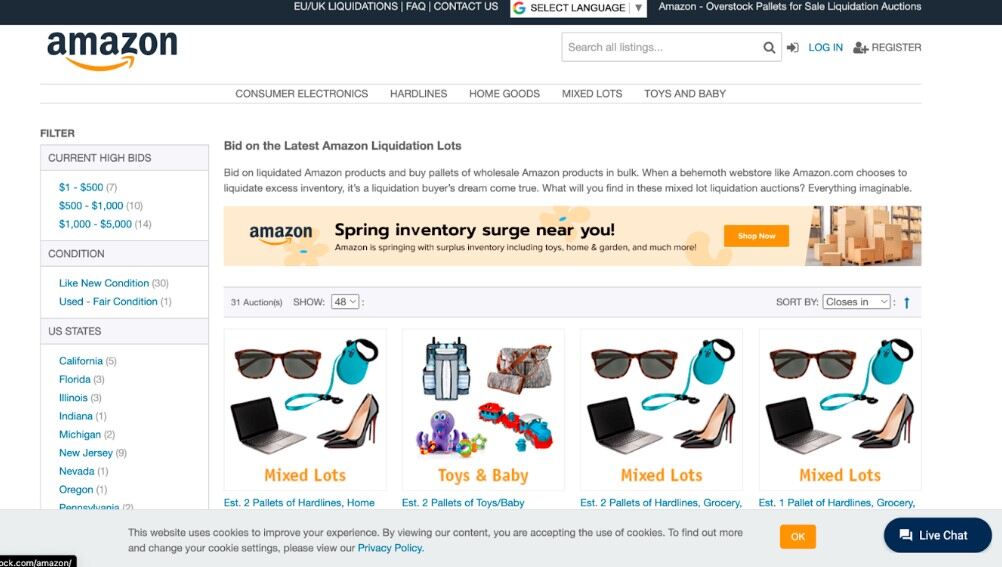**Detailed Caption:**

This screenshot captures an Amazon liquidation page displayed on a computer screen. At the very top of the page, a black navigation bar includes options such as "EU/UK Liquidations," "FAQ," and "Contact Us." Directly beneath this bar, there is a Google language selection icon followed by a drop-down box for selecting a language.

Centered prominently on the page is a headline that reads "Amazon Overstock Pallets for Sale: Liquidation Auctions," accompanied by the Amazon logo. The page is divided into several sections offering various types of auction lots including "Consumer Electronics," "Hard Lines," "Home Goods," "Mixed Lots," and "Toys & Babies."

On the left side of the screen, there are filter options for high bid amounts categorized into "$1 to $500," "$500 to $1000," and "$1000 to $5000." Additionally, the conditions of items are categorized as "Like New," "Used," and "Fair." Below these filters, different states are listed: California, Florida, Illinois, Indiana, Michigan, New Jersey, Nevada, and Oregon.

The right-hand side of the page features an invitation to "Bid on the latest Amazon Liquidation Lots," encouraging users to buy Amazon products in bulk, emphasizing the opportunities when a major retailer like Amazon liquidates surplus inventory.

A colored stripe on the page reads "Amazon Spring Inventory Surge Near You," promoting surplus inventory including toys, home and garden items, and more. A "Shop Now" call-to-action is included. Below this, there are 31 auction options displayed, primarily categorized as "Mixed Lots" and "Toys & Babies," each featuring images of potential items like sunglasses, high heels, computers, baby toys, and backpacks.

At the bottom of the page, a cookie consent notice appears, stating "This website uses cookies to improve your experience. By viewing our content, you are accepting the use of cookies. To find out more and change your cookie settings, please view our privacy policy," with an option to click "OK."